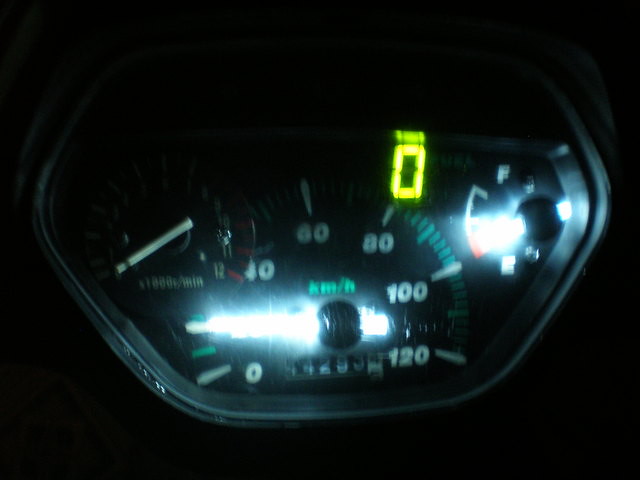This is a photograph capturing the dashboard of a car, specifically focusing on the speedometer. The photo’s quality is poor, likely taken at night or in a dimly lit environment, resulting in significant light reflections on the speedometer's plastic cover. These reflections manifest as white blobs in three distinct areas of the image, obscuring parts of the display. Despite the glare, the speedometer’s range is discernible, showing a scale from 0 to 120 kilometers per hour (km/h) in a turquoise font. Beneath the km/h indicator, there is a manually operated odometer displaying the vehicle’s mileage, although it is blurry and difficult to read, suggesting a figure over 14,000 miles. The rest of the dashboard features, including a dial in the upper left corner and a fuel gauge to the right of the speedometer, are significantly affected by the glare, making them nearly illegible.